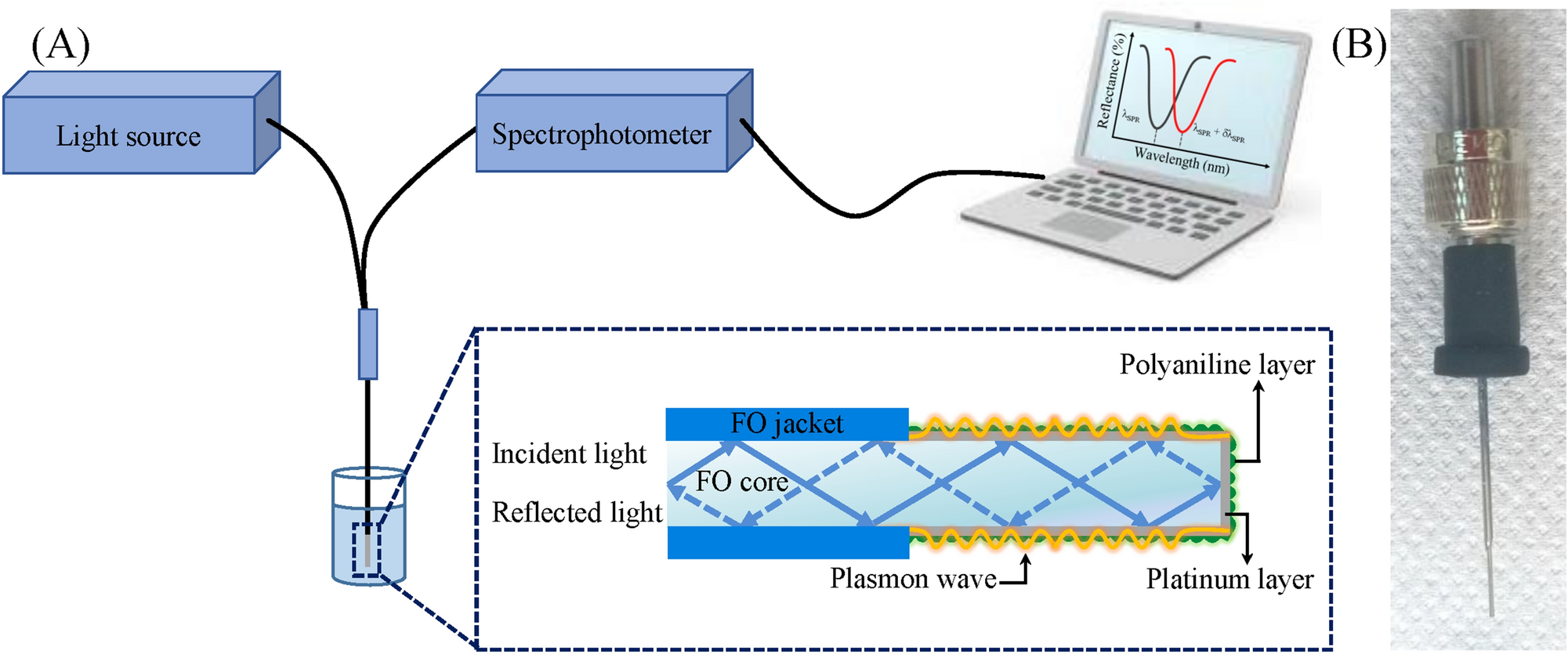The image is a detailed schematic diagram, blending hand-drawn elements with actual images, representing a scientific setup. The diagram is divided into sections labeled A and B.

In section A, the focal point is a blue, rectangular-shaped light source connected to a spectrophotometer, which is illustrated as another blue rectangle. This connection is shown through a cable or a black line, extending into a beaker filled with liquid. Inside this liquid is an expanded view with a blue-dotted rectangle, revealing the components: a foam (fo) jacket with an fo core, surrounded by layers of plasmon wave, platinum, and polyaniline. These intricate layers sit beneath the liquid surface. The spectrophotometer itself is connected via another cable to a laptop, which displays squiggly lines representing different reflectance wavelengths with annotations for incident and reflected light.

On the left-hand side of the laptop’s screen, details are provided through labels like "incident light", "reflected light", "plasmon wave", "fo core", and "fo jacket", while on the right-hand side, the labels "polyaniline layer" and "platinum layer" are noted. This setup is crucial for analyzing the spectra and providing wavelength data.

Section B showcases a different device featuring a sharp, needle-like tip, described as a thumbtack with an electrical element on top, labeled B. This part of the diagram contrasts the detailed setup of section A, providing context for another element involved in the scientific experiment.

Overall, the diagram serves as a comprehensive representation of the experimental setup, detailing the interaction between the light source, spectrophotometer, liquid medium with complex internal structures, and data collection via the laptop.